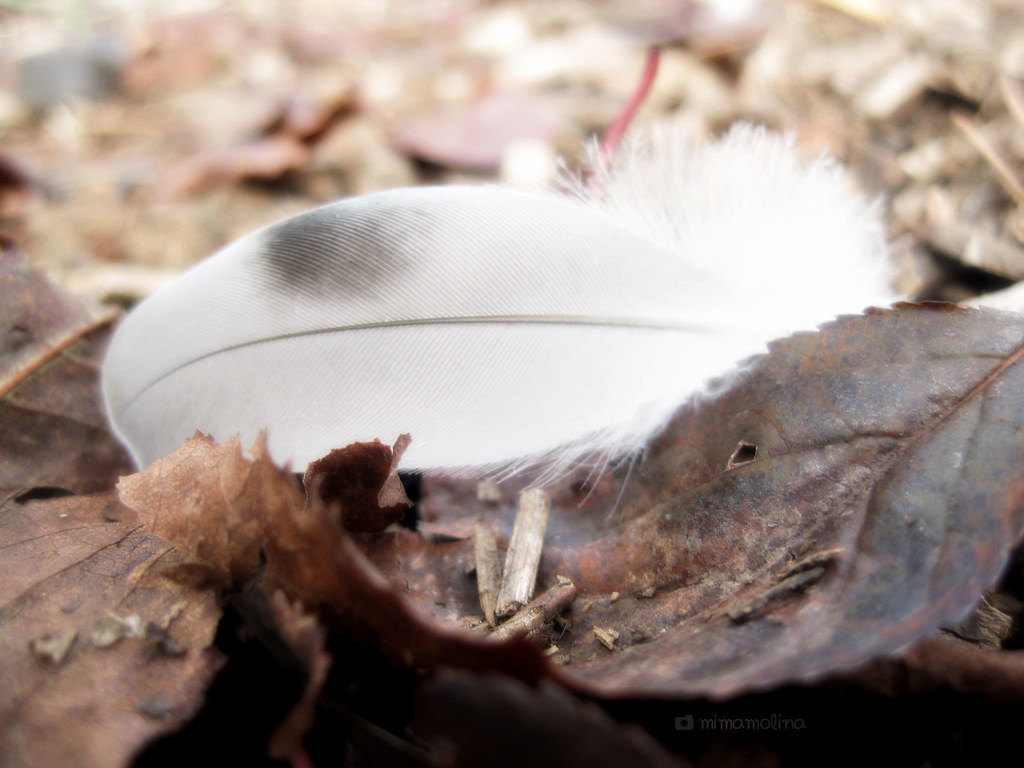This image captures an extreme close-up of the forest floor, where a single white feather rests delicately amidst a bed of dry, brown leaves. The leaves, some tinged with red and showing small holes, seem to have fallen recently, suggesting the scene is set in late autumn or early winter. Among the leaves, tiny broken sticks and pieces of wood can be seen, adding texture to the image. The feather, lying horizontally, features a distinct smudge of gray on its upper half and a tiny black mark, reminiscent of a thumbprint, at the very tip. Towards its base, the feather becomes soft, fluffy, and somewhat disheveled, resembling human hair. The background fades into a blur of more leaves and branches, drawing focus to the intricate details of the feather and the surrounding foliage. At the bottom of the photograph, there is an indistinguishable script, possibly the photographer's signature, though it is nearly illegible and difficult to determine if it is in the Latin alphabet. This focused vignette of nature offers a serene and introspective glimpse of the forest's floor.